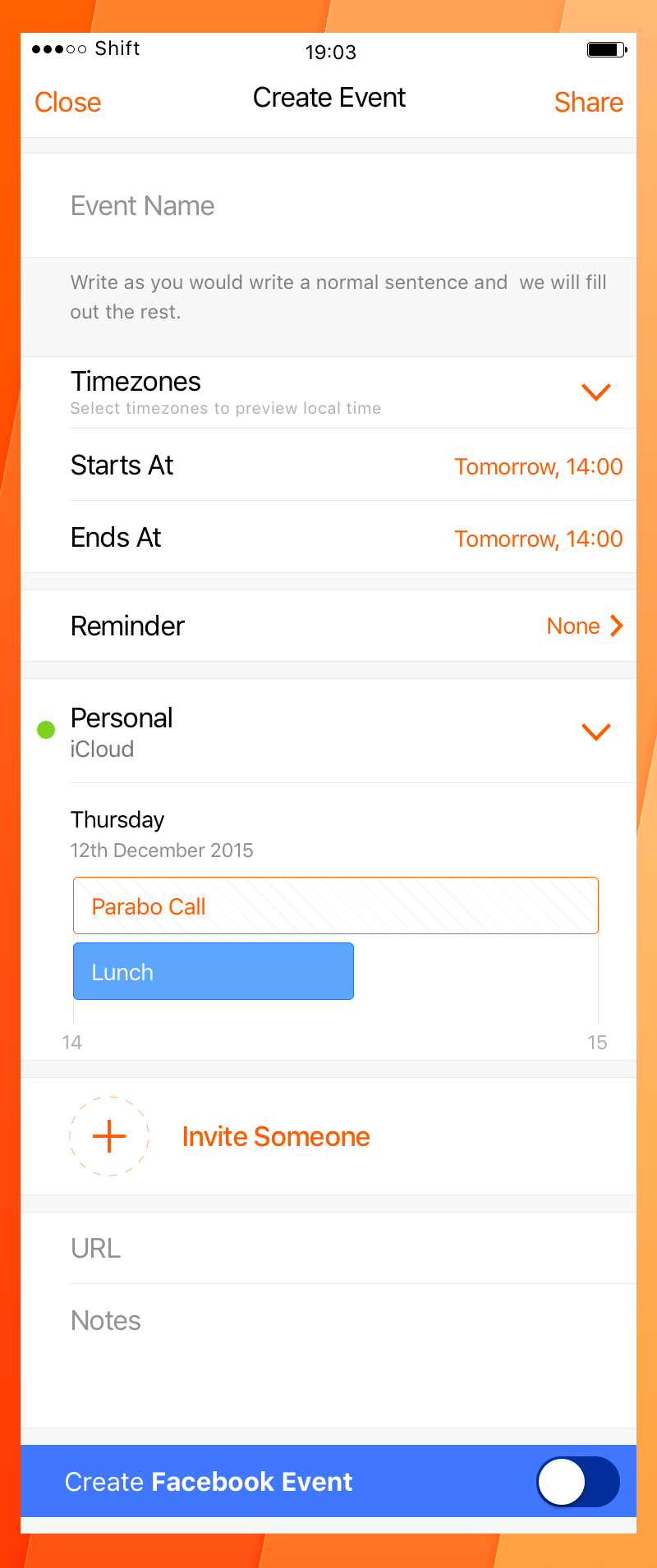This image captures a detailed screenshot taken on a mobile phone, clearly showing various elements of both the phone interface and an event creation screen within an app. 

**Top Section:**
- **Top-Left Corner:** Displays five horizontal dots indicating cell phone signal strength, with three dots filled in black and two remaining uncolored.
- **Top-Center:** Shows a timestamp reading "19:03."
- **Top-Right Corner:** Indicates the phone's battery percentage.

**Overall Appearance:**
- The screenshot is bordered by a gradient orange frame, which transitions from a darker orange on the left to lighter shades towards the right.

**App Interface:**
- The main content area indicates that the user is in an event creation mode within an app:
  - There are options to either close or share the event.
  - The space for typing an event name remains blank, signifying the initiation of a new event creation.
  - Below the event name field, a text prompt advises, "Write as you would write a normal sentence, and we will fill in the rest."

**Event Details Section:**
- Several customizable options are offered for setting event details:
  - **Time Zone:** Selection options for the event's time zone.
  - **Start and End Times:** Fields to specify when the event begins and ends.
  - **Reminder Settings:** Options to configure reminders for the event.
  - **Folder Selection:** Choices between placing the event in different folders, such as personal or iCloud.

**Additional Features:**
- A section dedicated to adding other options to the event, such as inviting participants and other customizable settings.

Overall, the screenshot showcases the interface of an event creation tool with a gradient orange border, clearly marked signal, time, and battery indicators, as well as various organizational features for scheduling and detailing an event.